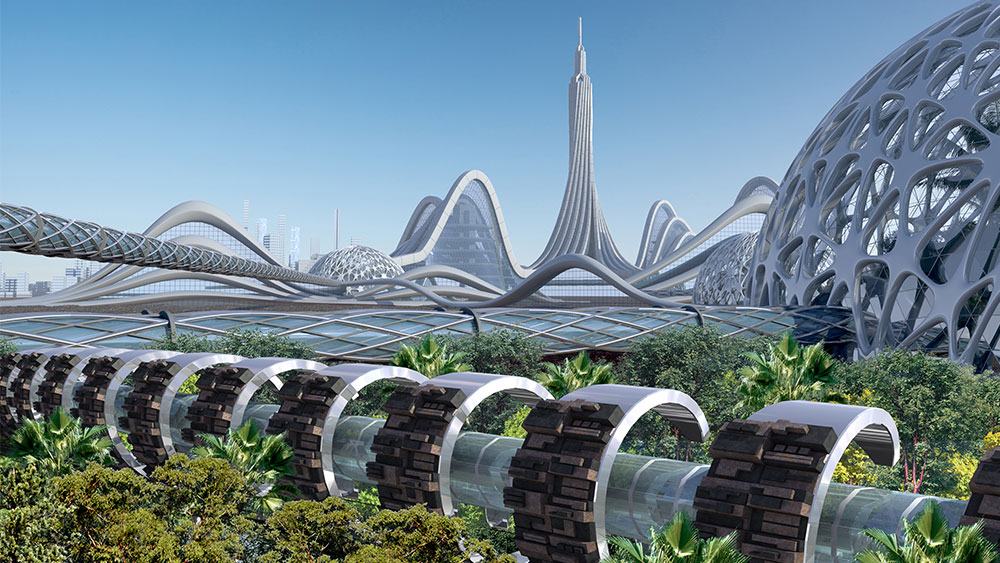The image depicts a futuristic urban landscape dominated by innovative architecture and lush greenery. In the foreground, vibrant green bushes and leaves create a natural base, contrasting with the complex structures above. A series of silver tubes traverse the scene, one prominently featuring a swirling, screw-like core wrapped by circular rings and adorned with irregular black elements. These tubes are intertwined with a network of curved arches, some resembling concrete filled with glass, suggesting an intricate transportation system.

To the right, a dome punctuated by triangular openings with smooth edges reveals glass beneath, adding to the futuristic aesthetic. Another dome can be seen farther in the distance. Standing tall in the center is a sophisticated tower, while the background is lined with modern, silvery blue skyscrapers. The scene is set under a clear, intensely blue sky, hinting at a meticulously designed, enclosed city environment that blends natural and artificial elements seamlessly. The overall impression is one of a highly advanced, three-dimensional cityscape ripe with unusual shapes and innovative design elements.